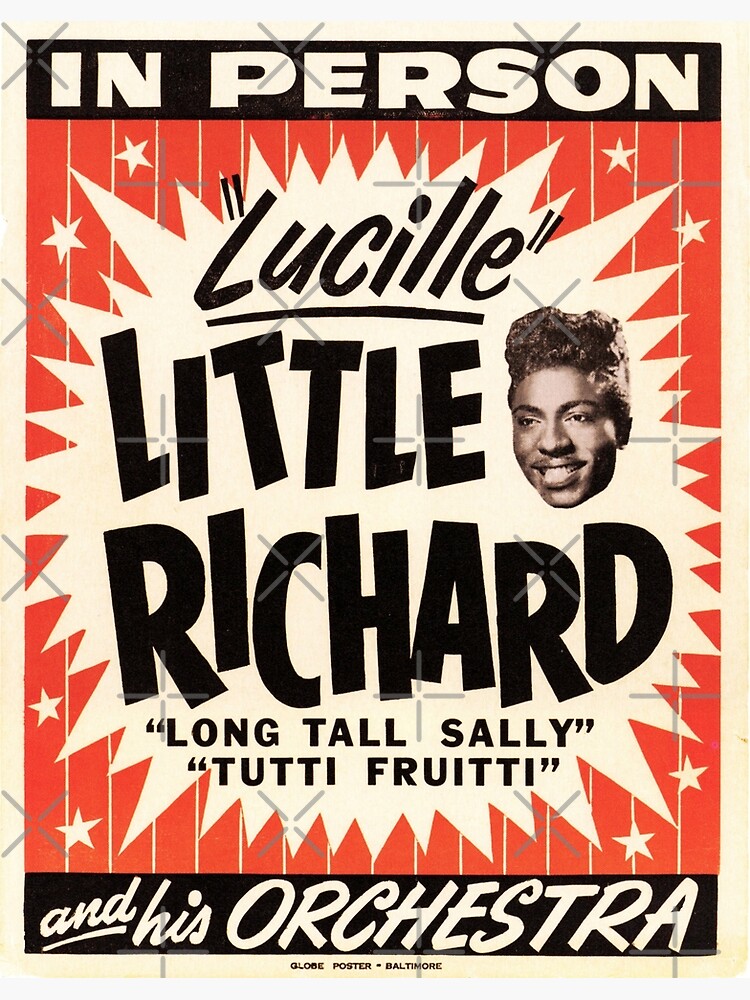This vintage-style poster features a vibrant red background with borders adorned by stars. At the top, a black band displays the phrase "In Person" in bold white letters. Below this, against a white burst background with spiky edges, the names of Little Richard's iconic songs are listed: "Lucille," "Long Tall Sally," and "Tutti Frutti," all in black font. To the left of these titles is a black-and-white image of Little Richard's smiling face. At the bottom, another black band contains the text "and his orchestra." The overall design evokes a classic, nostalgic feel, celebrating the legendary musician and his timeless hits.